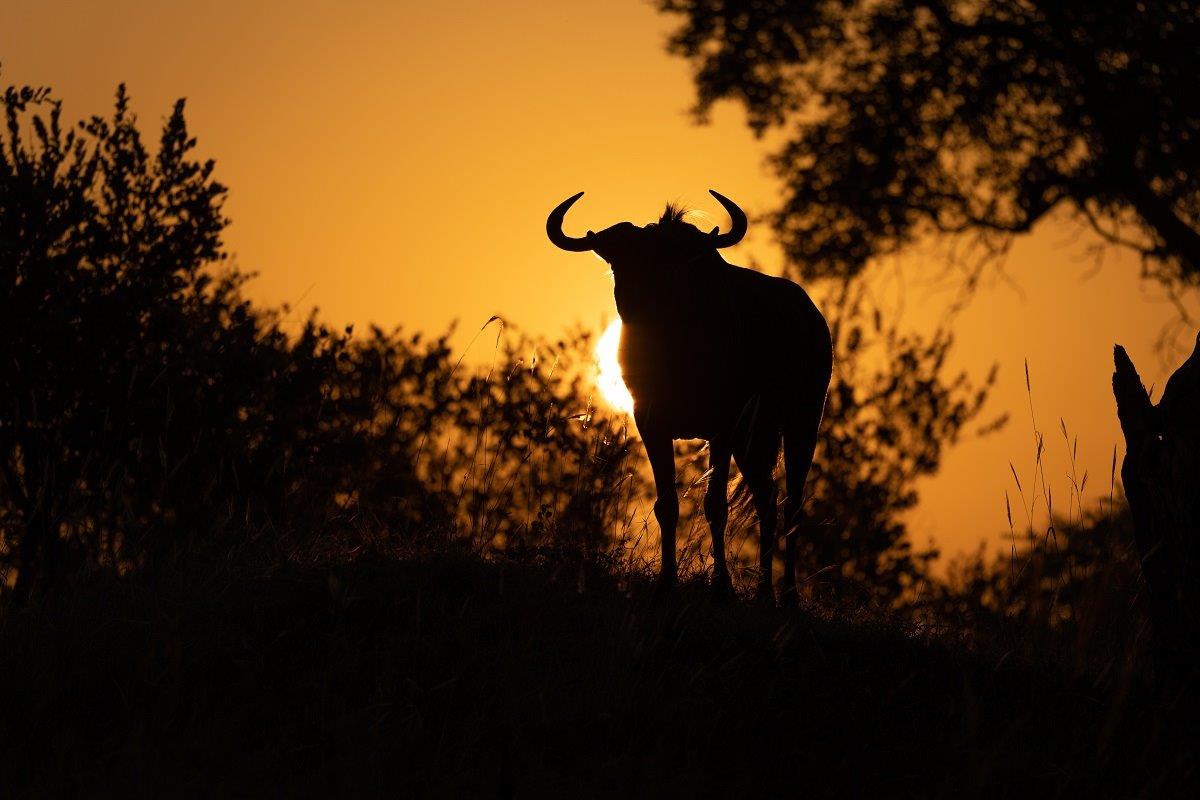The photograph captures a dramatic sunset, with the sky glowing in vibrant shades of yellow and orange, transitioning to a duller hue at the edges. The sun, resembling a yellow ball, sits directly behind a silhouetted animal, likely a buffalo or a wildebeest, casting it into profound shadow. This animal's distinctive curved horns and tall, thin legs are prominently outlined against the setting sun. The animal stands amidst tall grass, weeds, and brush, blending into the shadowed left side of the image. To the right, a tree trunk with a short branch sticks out, and more tree branches lean to the left from the top right corner. Black shadows from bushes add depth to the foreground, and the distant hills seem to meld together in the dimming light. The composition conveys a peaceful yet powerful scene that accentuates the wild beauty of the landscape at dusk.